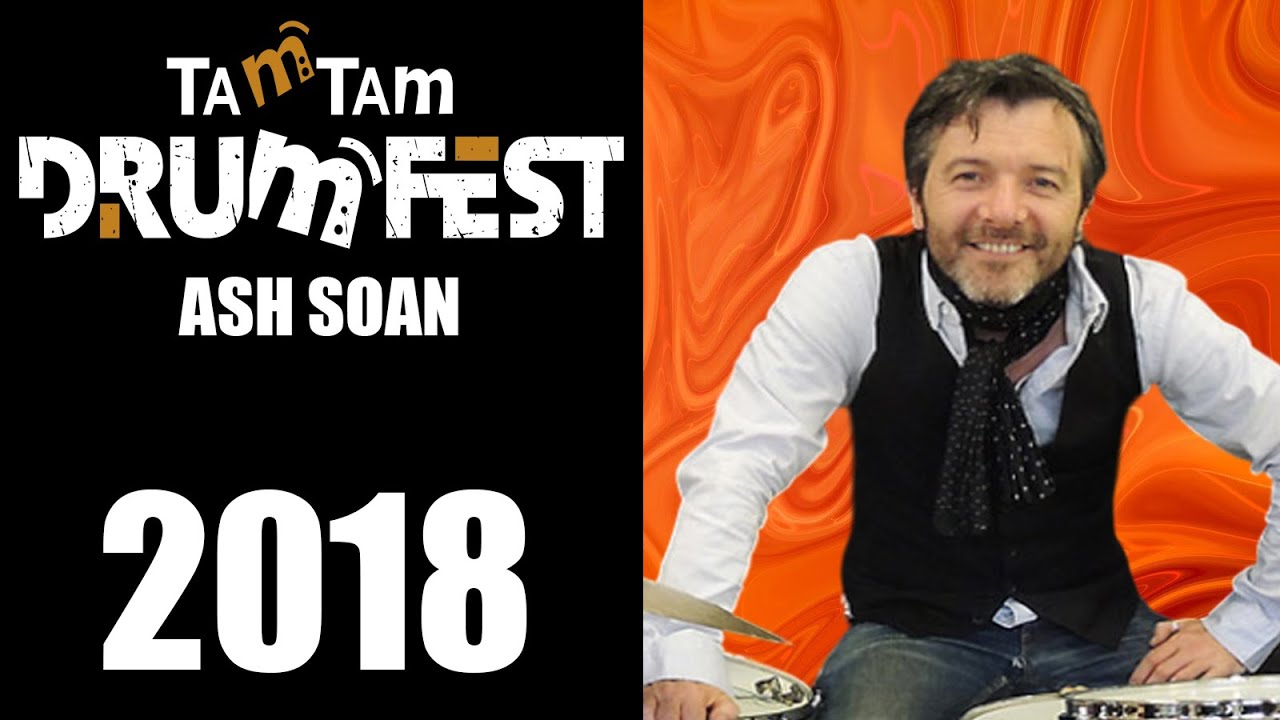The rectangular image measures about six inches wide by three inches high and is divided into two distinct sections. The left side features a plain black background with stylized white and brown text. At the top, "Tam Tam Drum Fest" is printed in white, except for the first "M" in "Tam Tam," which is raised and colored brown, and the first leg of the "R" in "Drum," also brown. The "E" in "Fest" has its top stripe colored brown. Beneath this, the event name "Ash Soan" is displayed in white letters. The right side of the image is a photograph of a Caucasian man with short brown hair speckled with gray. He has a smiling face with a visible top row of teeth, a brown mustache, and a graying beard. He is dressed in a long-sleeve white shirt, a black vest, a black neckerchief, and blue jeans. The man appears to be leaning slightly on a drum set, set against a wavy orange curtain backdrop. The overall composition juxtaposes the stylishly designed event information with the friendly, approachable image of the drummer, Ash Soan.